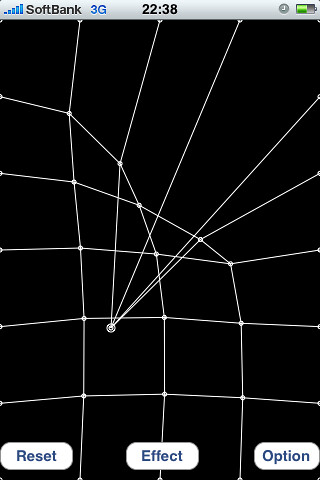The image is a detailed smartphone screenshot, evident by the display of typical phone indicators at the top. The top banner, a light grayish-silver color, shows five blue signal bars next to the black text "SoftBank" followed by a blue "3G." Centered at the top is the time "22:38" in black text. To the right, a gray clock icon suggests an alarm is set, and further right, the battery indicator is half full, marked by a green bar.

The main portion of the image features a complex geometric grid in black and white, resembling a distorted set of vector graphics with lines connecting various points, creating shapes like squares and triangles. This grid seems to have been manipulated, as if sections have been dragged out of place.

At the very bottom, three oval-shaped buttons with blue text on gray backgrounds are labeled "Reset" on the left, "Effect" in the middle, and "Option" on the right. This image gives the impression of a creative or technical interface likely used for some form of graphic editing or manipulation.